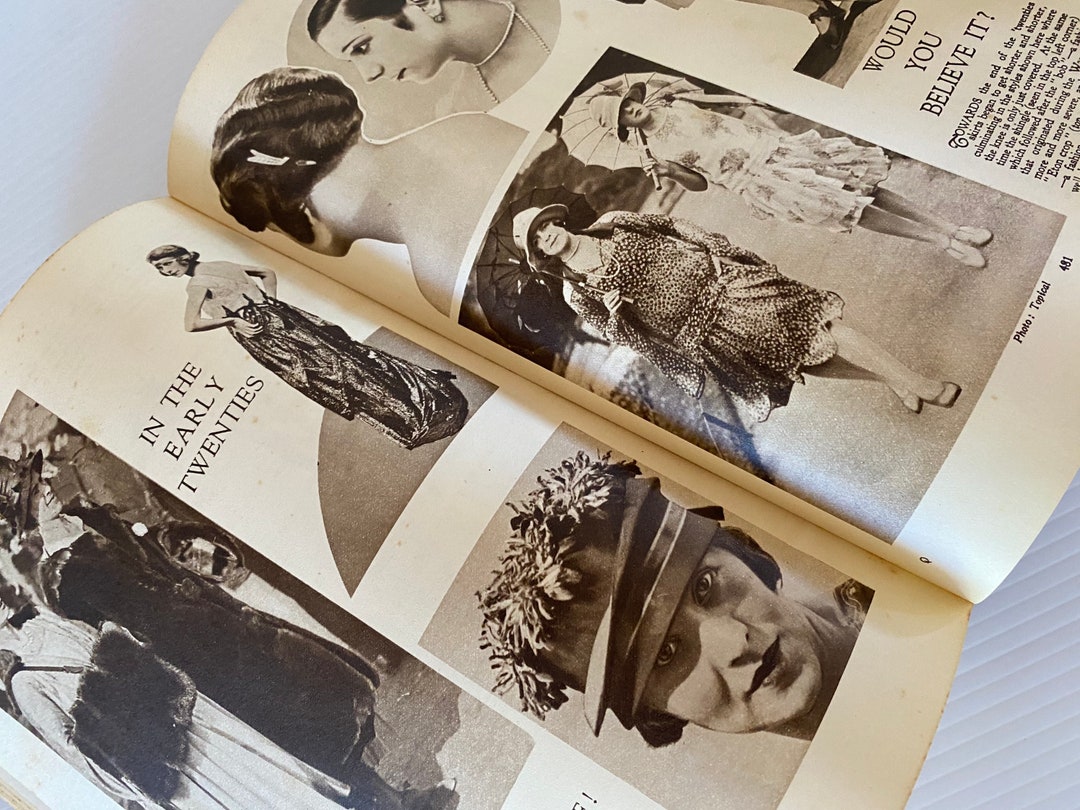The image, an indoor color photograph of an open black-and-white magazine, captures a nostalgic portrayal of 1920s fashion and hairstyles. On the left page, several images depict women in various stages of dress. There is a collage of outfits, including a woman in a long fur coat with a matching handbag behind her, and another woman in a strapless dress that flows to the ground, labeled "in the early 20s." The bottom of this page features a close-up of a woman's face adorned with a hat decorated with flowers, covering her eyebrows. 

On the right page, the focus is on a woman’s elegant updo hairstyle, complemented by a necklace. Below this, two women are displayed side-by-side, dressed in flapper-style dresses, with hats resting over their eyebrows and parasols draped over their shoulders. The magazine offers a glimpse into early 20th-century women's attire, complete with silent movie star-style hairdos and floral hats, creating a rich, old-fashioned atmosphere further enhanced by accompanying text that reads "in the early 20s" and "would you believe it?"